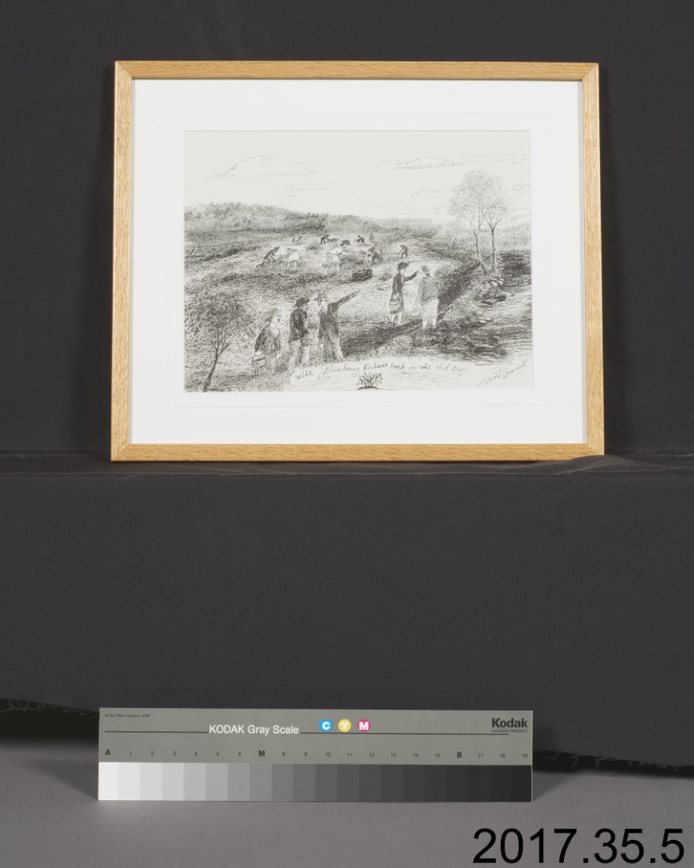The image depicts a photograph of a framed black and white sketch, elegantly situated against a dark gray background. The artwork, confined within a light-colored wooden frame, is presumably a pencil drawing of an old-fashioned rural scene, reminiscent of pilgrim times. The illustration captures an outdoor landscape, featuring several figures who appear to be farming or tending to fields, with a small hill or wall running through the center and off into the distance. Trees sporadically dot the landscape, adding to the pastoral feel. 

Beneath the framed picture lies a Kodak grayscale strip, which appears to be a three-dimensional object. This grayscale is rectangular, with smaller rectangles transitioning from bright white to deep black from left to right, accompanied by letters above each segment. The strip includes colored dots, likely representing cyan, yellow, and magenta. Notably, the bottom right corner of the grayscale displays the sequence “2017.35.5,” which could be an identifier rather than a date. The grayscale and the artwork collectively sit on a ledge that matches the wall's color, subtly blending into the background.